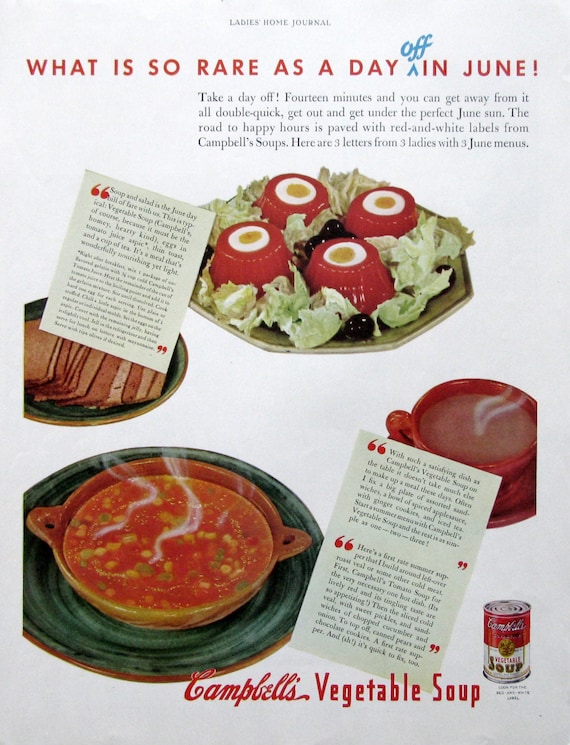This image features a vintage advertisement from the Ladies' Home Journal promoting Campbell's Vegetable Soup with the headline, "What is so rare as a day off in June?" The ad suggests taking a brief, 14-minute escape to enjoy the perfect June sun, indicating the ease and quick preparation of the soup. The tagline reads, "The road to happy hours is paved with red and white labels from Campbell's Soups."

The advertisement showcases three letters from women sharing quick and easy June menu ideas, which are ideal for those looking to maximize their leisure time during a day off. The visual elements include a prominent bowl of vegetable soup set on a green plate, displaying visible pieces of vegetables. Beside it, there is a cup believed to contain coffee, and additional food items on the table include a jello-like salad adorned with olives and lettuce, as well as a plate of bread or crackers. In the bottom right corner, there is also an image of a Campbell's Soup can. The combination of these elements emphasizes the variety and convenience of meal options using Campbell's Vegetable Soup.